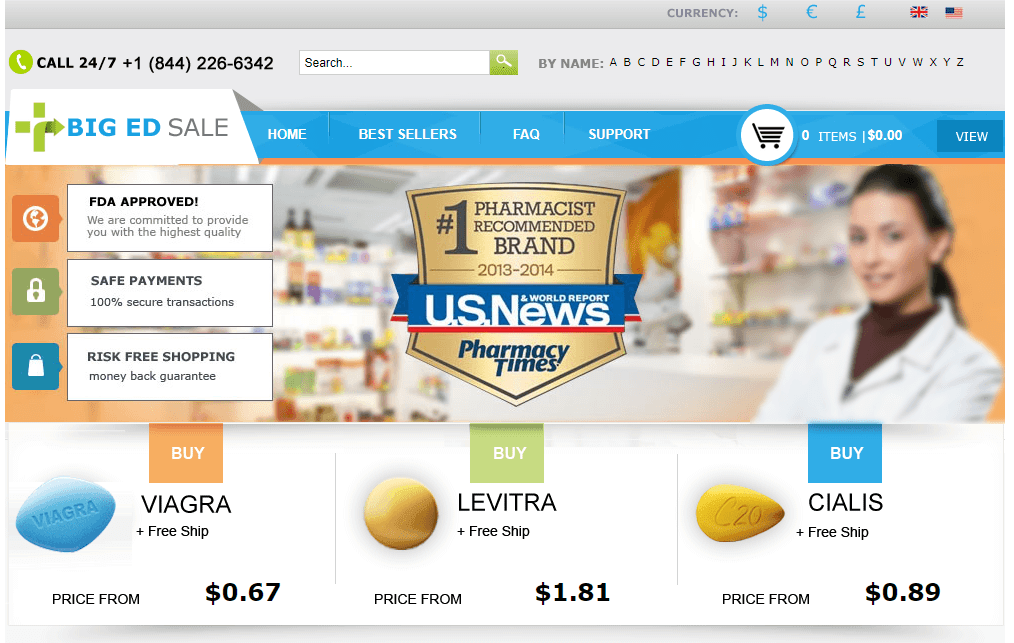This image showcases a detailed view of a pharmacy website. The background is light gray or white, and at the very top of the site, there's a thin, darker gray bar. On the left side of this bar, the word "Currency" is displayed in gray text, along with symbols for the dollar, pound, and euro. On the right side of this bar, the British and American flags are shown. 

Below this bar, moving from the top left to the right, there is a green circle with a white telephone icon inside it and a black text that reads "Call 24/7 +1 844 226 6342." Next to it, there's a white search bar with a green search button, labeled "By Name," followed by the letters A through Z.

In the middle of the website, a large banner displays a blurry image of a typical pharmacy counter with a woman pharmacist in the background. The text on the banner reads, "Big Ed Sale," and a light blue sub-banner contains navigation options: "Home," "Bestsellers," "Back," and "Support," as well as a shopping cart icon showing "0 items $0 View."

Beneath this, several phrases are listed prominently: "FDA Approved," "Safe Payments," and "Risk-Free Shopping." A gold shield in the center states "Number One Pharmacist Recommended Brand 2013-2014, US News and World Report, Pharmacy Times."

At the bottom of the image, three pills are displayed: a blue pill labeled "Viagra," a circular yellow pill labeled "Levitra," and a yellow pill inscribed with "C20" labeled "Cialis." The respective prices are from $0.67, $1.81, and $0.89. The words "Buy" and "Free Ship" are also noted.